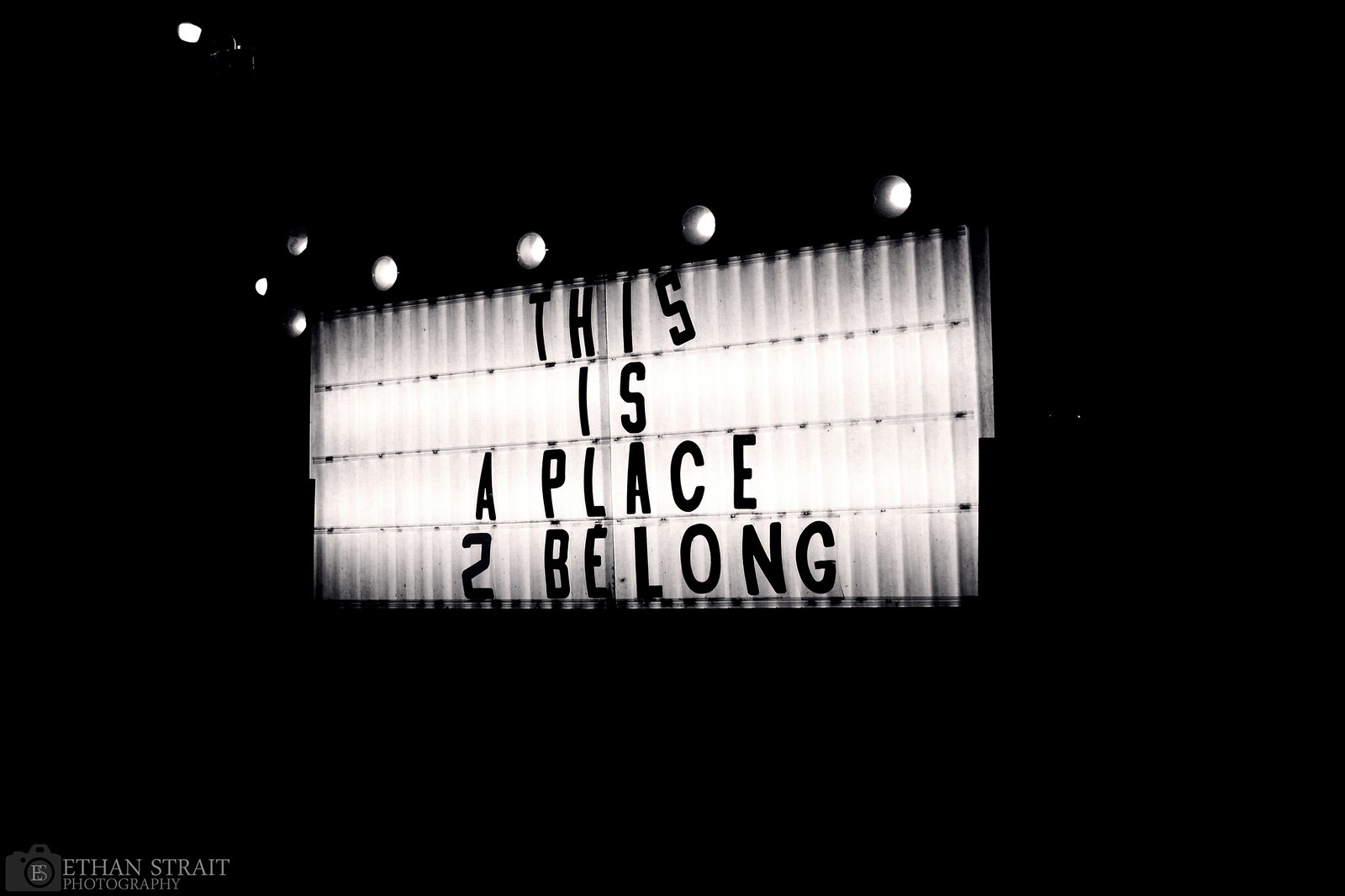The black-and-white photograph captures a minimalistic scene dominated by darkness, with the focal point being an illuminated outdoor sign typically seen at bars or restaurants. The self-lit sign, featuring a retro letterboard where phrases can be customized, prominently displays the message "This is a place 2 belong," with the number "2" replacing the word "to." The sign's backdrop is a clear plastic plate, allowing the backlit letters to stand out vividly against the surrounding blackness. 

At the top of the sign are light bulbs arranged to form an arrow pointing left, reminiscent of marquee lights, suggesting movement or direction towards a venue. Another distant streetlight is faintly visible in the upper left corner of the image, adding a subtle gradient to the overall grayscale tone.

The photograph includes a detailed watermark in the bottom left corner, featuring an icon of a camera and the text "Ethan Straight Photography," attributing the image to its creator. The rest of the image remains pitch-black, emphasizing the glowing sign as the central element.